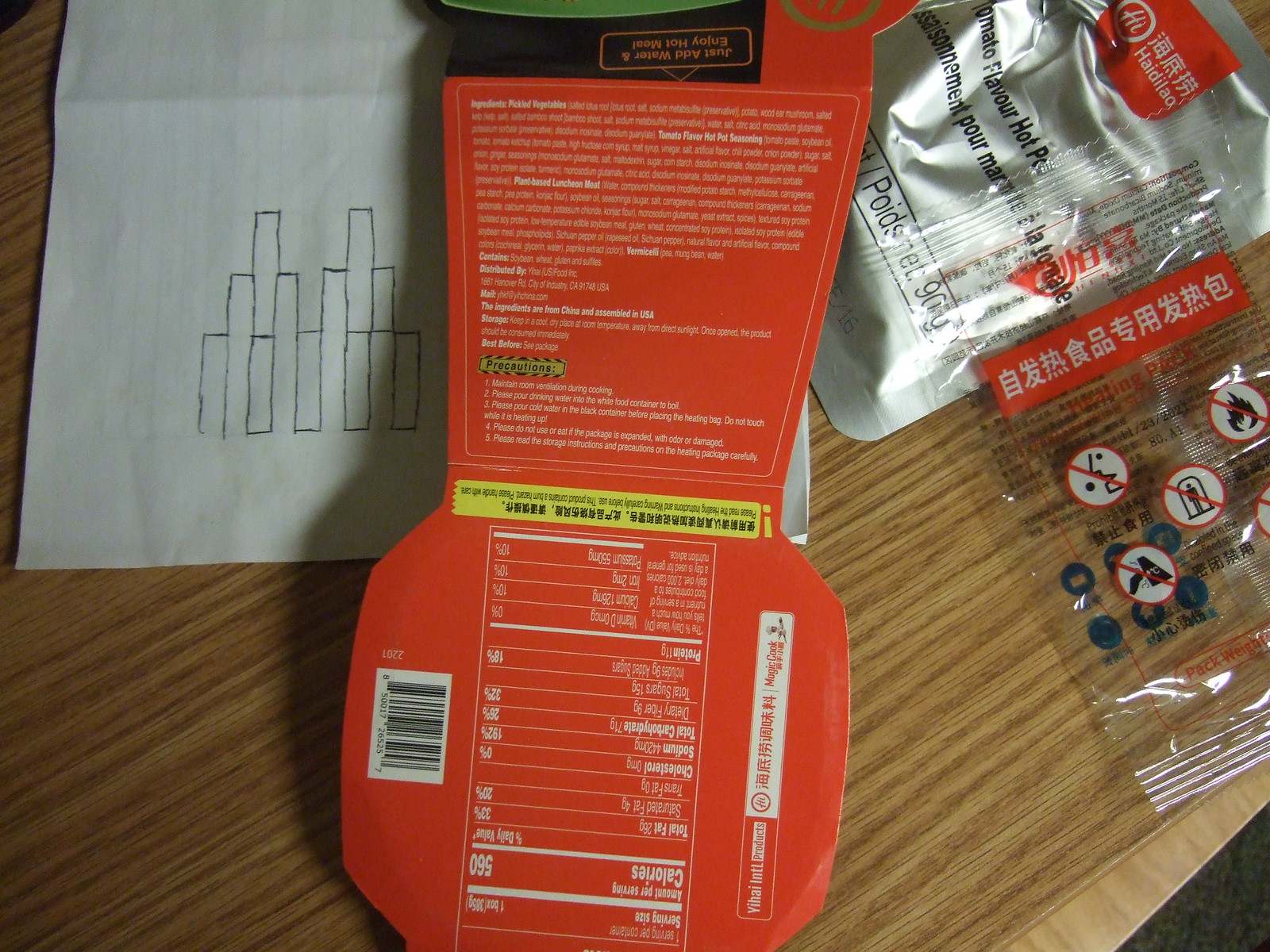The image is a photograph of food product packaging displayed on a wooden table. Multiple packets, all related to the same tomato-flavored hot pot instant meal, are laid out flat. The packaging features writing in what appears to be Chinese characters, though the image quality makes reading finer details difficult. Visible information on the packaging includes ingredients, serving instructions, and nutritional data. A white piece of paper with black, block-shaped bars drawn on it is partially visible beneath the packets, adding an additional element of interest to the composition.